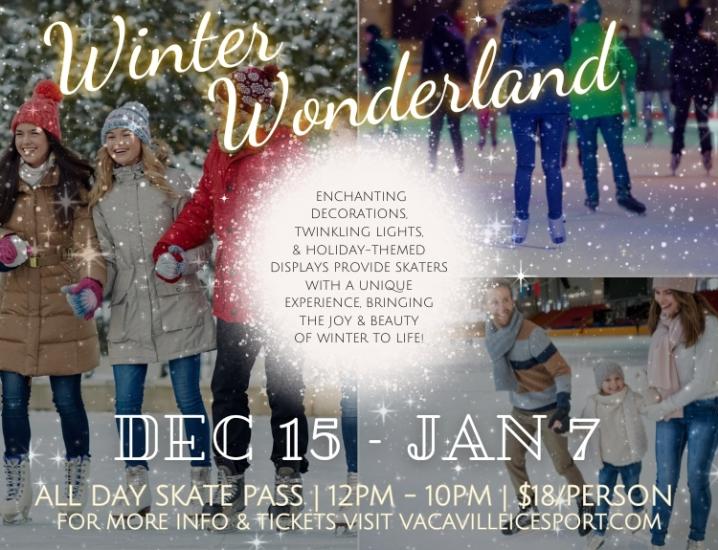This is a horizontal rectangular advertisement designed for an event titled "Winter Wonderland," displayed at the top in light yellow cursive writing. The image backdrop features three photographs of people in winter jackets and jeans, enjoying ice skating outdoors amidst decorations and snow-covered Christmas trees. A larger photograph occupies the left side, showing a bustling ice skating rink, while two smaller images on the right capture joyful skaters having fun.

At the center of the advertisement is a glowing white starburst with sparkles and snowflakes, overlaying text that reads: "Enchanting decorations, twinkling lights, eight holiday-themed displays provide skaters with a unique experience, bringing the joy and beauty of winter to life." Below this, additional details are provided: the event runs from December 15th to January 7th, with all-day skate passes available from 12 p.m. to 10 p.m. at $18 per person. For more information and tickets, visitors are directed to visit vacavilleicesport.com.